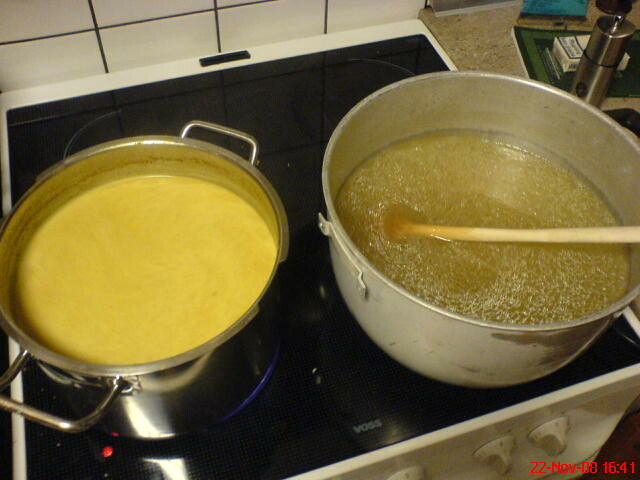This color photograph, taken on November 22, 2008, at 16:41, showcases a black Voss brand stovetop, viewed from above. The stovetop's dials are white and plastic-looking, positioned on the front panel. Surrounding the stovetop, a backdrop of white tiles is visible. On the left sits a large metal pan with handles, containing a thick, viscous, yellow liquid, possibly a creamy soup or roux. To the right, an even larger silver-colored saucepan holds a soup with a visible layer of fat, suggesting a broth, potentially chicken. Alongside the stove, there are various ingredients and what appears to be a packet of cigarettes placed on the countertop. The overall image is slightly unclear, but the main elements are identifiable, capturing a home-cooking scene in progress.